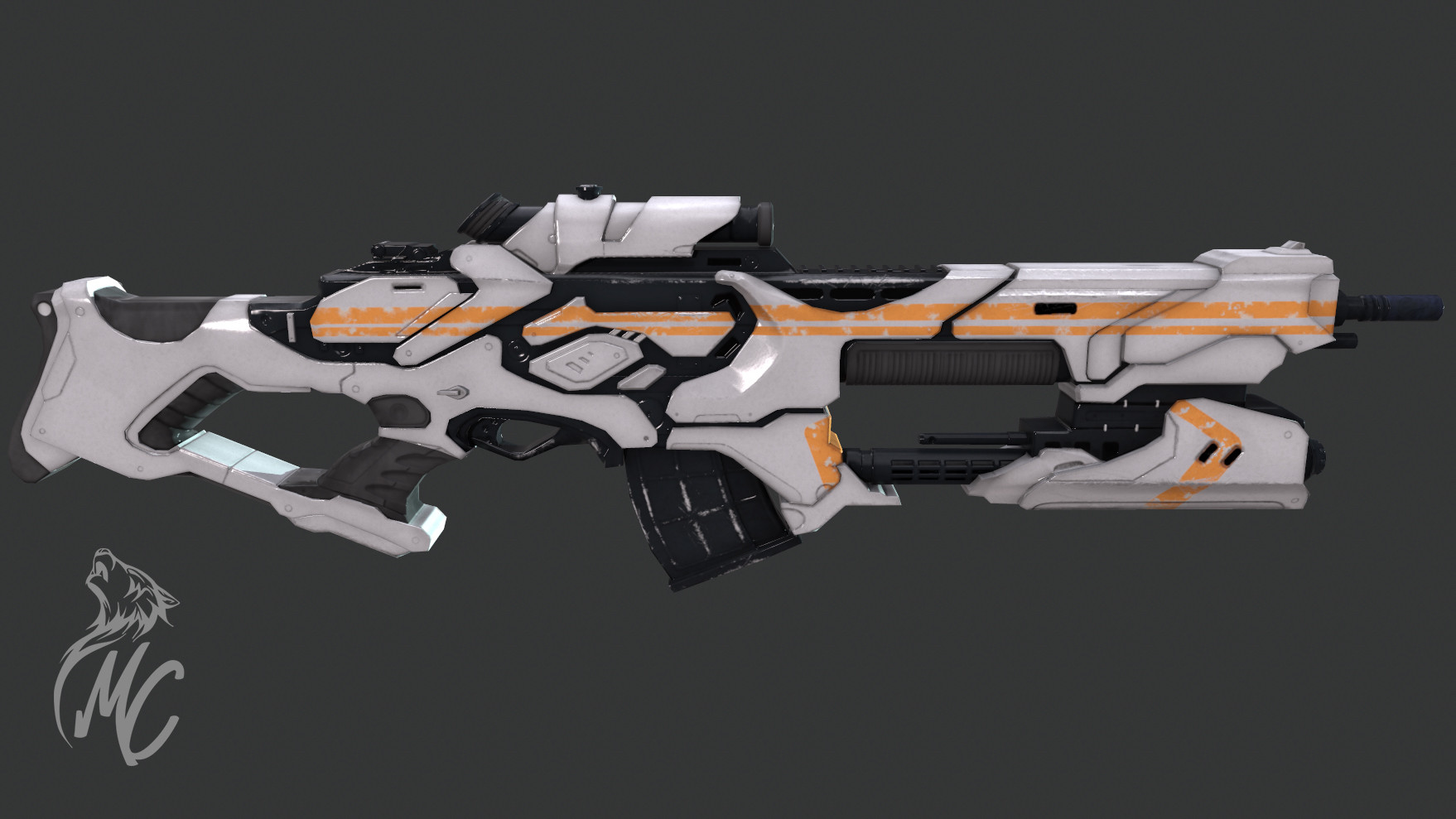The image displays a highly detailed, 3D rendering of a futuristic, science fiction gun. Positioned within a horizontally rectangular frame with a solid, slate-gray background, the gun's barrel is oriented towards the right side while the buttstock faces left. Dominantly white with striking orange stripes that run from back to front, the gun features a sleek, space-age design.

Notable elements include a black, forward-curving magazine attached at the bottom, and a robust, black scope set atop the barrel within a white casing. The trigger guard is distinctly square-shaped. The stock, connected via a white section, sports a visually gripping design and an ergonomic grip.

In the image’s lower left corner sits the artist’s watermark: a gray text "MC" alongside a stylized wolf’s head howling upwards. The watermark, shaped to resemble brush strokes, subtly blends into the dark gray background, adding a signature aesthetic.

The composition and digital enhancements lend the gun a realistic, yet fantastical appearance, evoking a high-tech, space-faring narrative familiar in contemporary science fiction, or potentially as a modernistic toy.